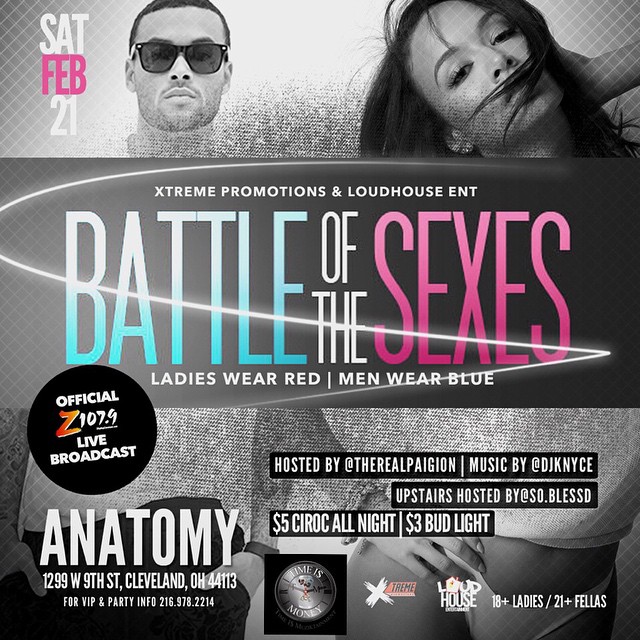The promotional flyer for the "Battle of the Sexes" event, hosted by Extreme Promotions and Loud House Entertainment, features a visually striking design with key details prominently displayed. At the top center, in bold letters, it announces the event, with "Battle of the Sexes" highlighted in large pink and blue font. The background showcases dramatic, bright curving lights sweeping across the image. To the left is a serious-looking man wearing dark-rimmed large sunglasses, while on the right, a woman strikes a sexy pose with her hand behind her head and her hair flowing.

The event is set to take place on Saturday, February 21st, and specifies the dress code: ladies wear red and men wear blue. The bottom left of the flyer details the venue information: Anatomy Gentlemen's Club at 1299 West 9th Street, Cleveland, Ohio, 44113. A live broadcast will be provided by Z107.9. For VIP and party info, a contact number is provided: 216-978-2214.

Additional event details include:
- Hosted by The Real Paigion and music by DJ KNYCE.
- Upstairs hosted by So Blessed.
- Drink specials: $5 Ciroc all night and $3 Bud Light.
- The flyer also indicates age restrictions: 18+ for ladies and 21+ for men.

This vivid and comprehensive flyer ensures attendees are well-informed about the "Battle of the Sexes" at the Anatomy Gentlemen's Club, promising a lively and exciting event.